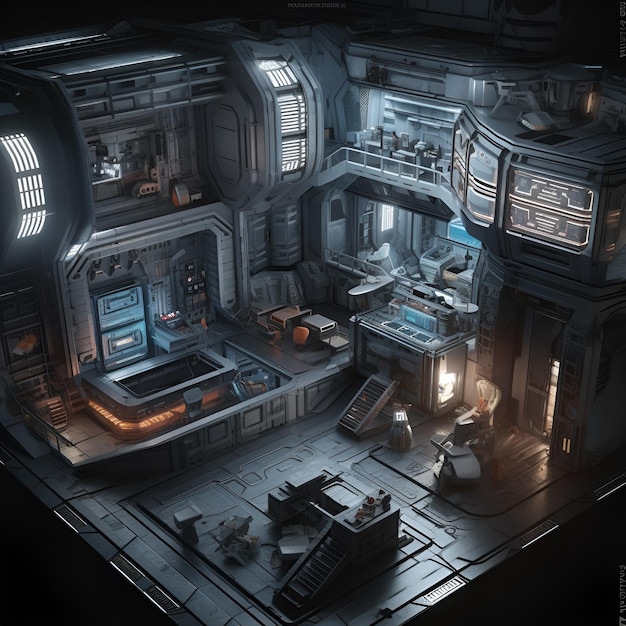The image is a highly detailed, computer-generated interior of a futuristic dwelling or command center reminiscent of a setting from a sci-fi movie, potentially "Star Wars" or "The Matrix." Predominantly rendered in various shades of gray, the space is illuminated by bright yellow lights integrated into hexagonal patterns on the upper levels. The structure spans multiple levels, interconnected by ladder-like steps and small stairwells. The environment is devoid of people but is filled with a plethora of machinery and technological equipment, giving the impression of an advanced lab or monitoring station. Various seating areas with chairs suggest the presence of workstations rather than sleeping quarters. The space appears optimized for labor and technical operations, featuring multiple illuminated sections that imply active technological processing and monitoring. The entire setting may also resemble the interior of a colossal machine or a command hub from a high-tech video game, further emphasizing the blend of futuristic aesthetics and intricate design elements.